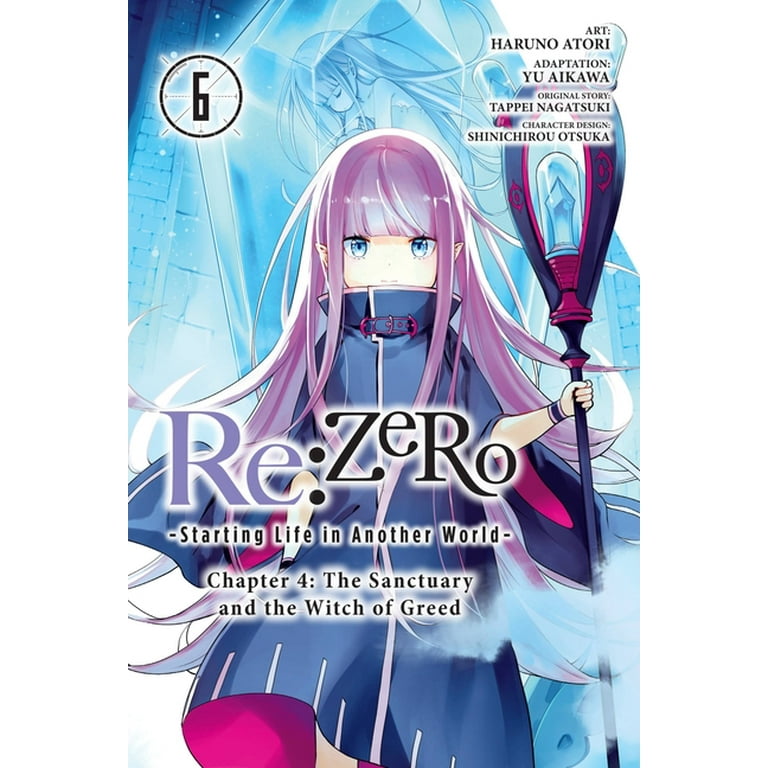This image is a highly detailed, color illustration that appears to be the cover of a manga titled "Re:Zero - Starting Life in Another World, Chapter Four: The Sanctuary of the Witch of Greed." Centered prominently on the cover, the title features "Re" in purple letters and "Zero" in black, with the subtitle below in black text on a white background. Above the title, in the left corner, a number six is enclosed within a clock-like design.

The central figure is a young elf girl with long pink hair and blue eyes, dressed in a long blue trench coat with a raised collar accented with pink details. She holds an elaborate staff with a crystal in the center of a ring-shaped top, which is adorned with two additional crystals. Her light pale skin and pointed ears further highlight her elf-like features.

In the background, another girl who closely resembles the elf is depicted encased in a large blue crystal in a fetal position. The overall background is light blue, enhancing the ethereal and magical atmosphere of the scene. The cover combines intricate character details and mystical elements, creating an engaging and dramatic visual presentation.